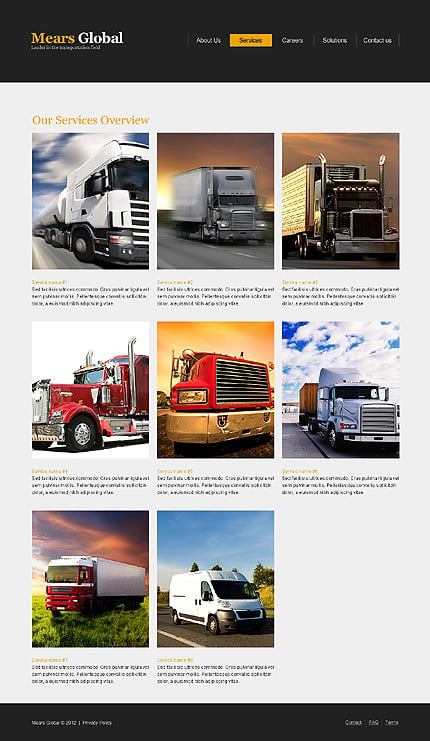The image features the homepage of a website called "Mears Global." The site's name, "Mears Global," appears on the left side of the header, with "Mears" in yellow-gold text and "Global" in white. Positioned to the right are navigation links, including "About Us," "Services," "Careers," "Solutions," and "Contact Us," with "Services" highlighted by a gold bar and black text, indicating it is the selected section.

Centered below the navigation links is an orange header reading "Our Services Overview." Beneath this header are eight photographs, all depicting various trucks. The top row displays three white trucks, seemingly in transit on a roadway. The middle row features two red trucks and one light blue truck; the blue truck is parked against a backdrop of a blue, cloudy sky, while one of the red trucks is captured at sunset. The bottom row showcases a red and white truck and a smaller vehicle that appears more like a van, with the red and white truck stationed on the grass.

Each photo is accompanied by paragraphs of information, too small to be legible. The page concludes with a black bar containing white text.